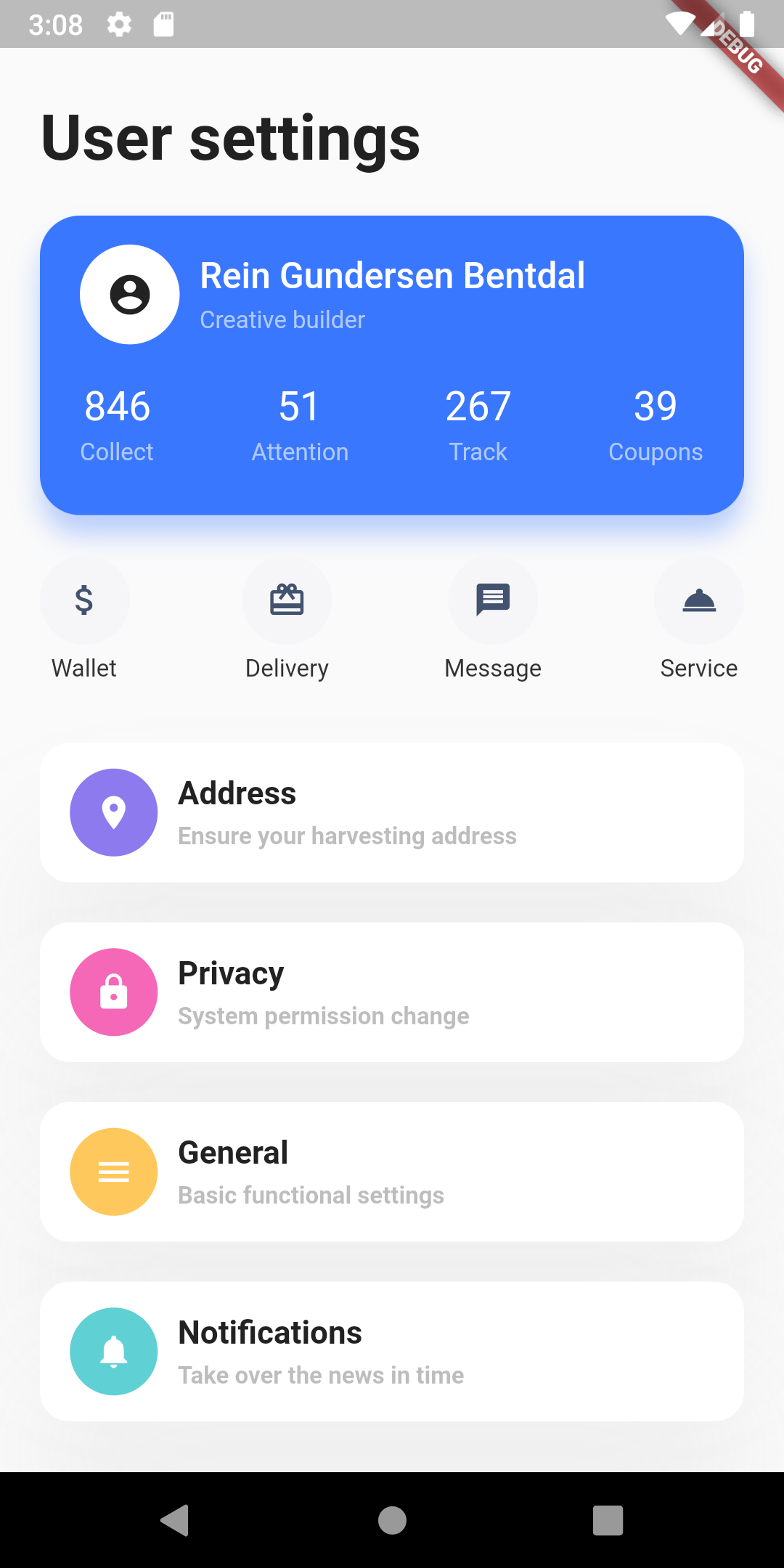### Detailed Caption for the Screenshot

The image depicts a phone screen displaying the "User Settings" section under "Web Settings". The time displayed is 3:08, but it is unclear if this is AM or PM. 

At the top of the screen, there is a Settings icon alongside a lock icon. The battery indicator shows a full charge, and Wi-Fi is enabled. A prominent red line crosses one corner of the screen with the word "Debug" written on it.

Below the "User Settings" title, there's a blue rectangular box containing the name "Rain Gunderson Benthal" along with the designation "Creative Builder". Beside the name, there's a standard profile icon featuring a white circle with a black center, indicating that no custom profile image has been set.

Underneath the profile information, various activity statistics are displayed:
- **846** labeled as "Collect"
- **51** labeled as "Attention"
- **267** labeled as "Track"
- **39** labeled as "Coupons"

Following these statistics, there are four clickable options: "Wallet and Delivery," "Message and Service," each listed consecutively.

Further down, the screen shows:
- **Address** with a map icon
- A prompt stating, "Ensure your Harvesting Address"
- **Privacy** indicated by a lock icon within a pink circle
- **System Permission Change**
- **General** represented by three horizontal bars
- **Basic Functional Settings**
- **Notifications** accompanied by a bell icon

This comprehensive setup implies a robust set of user options tailored for advanced personalization and management.